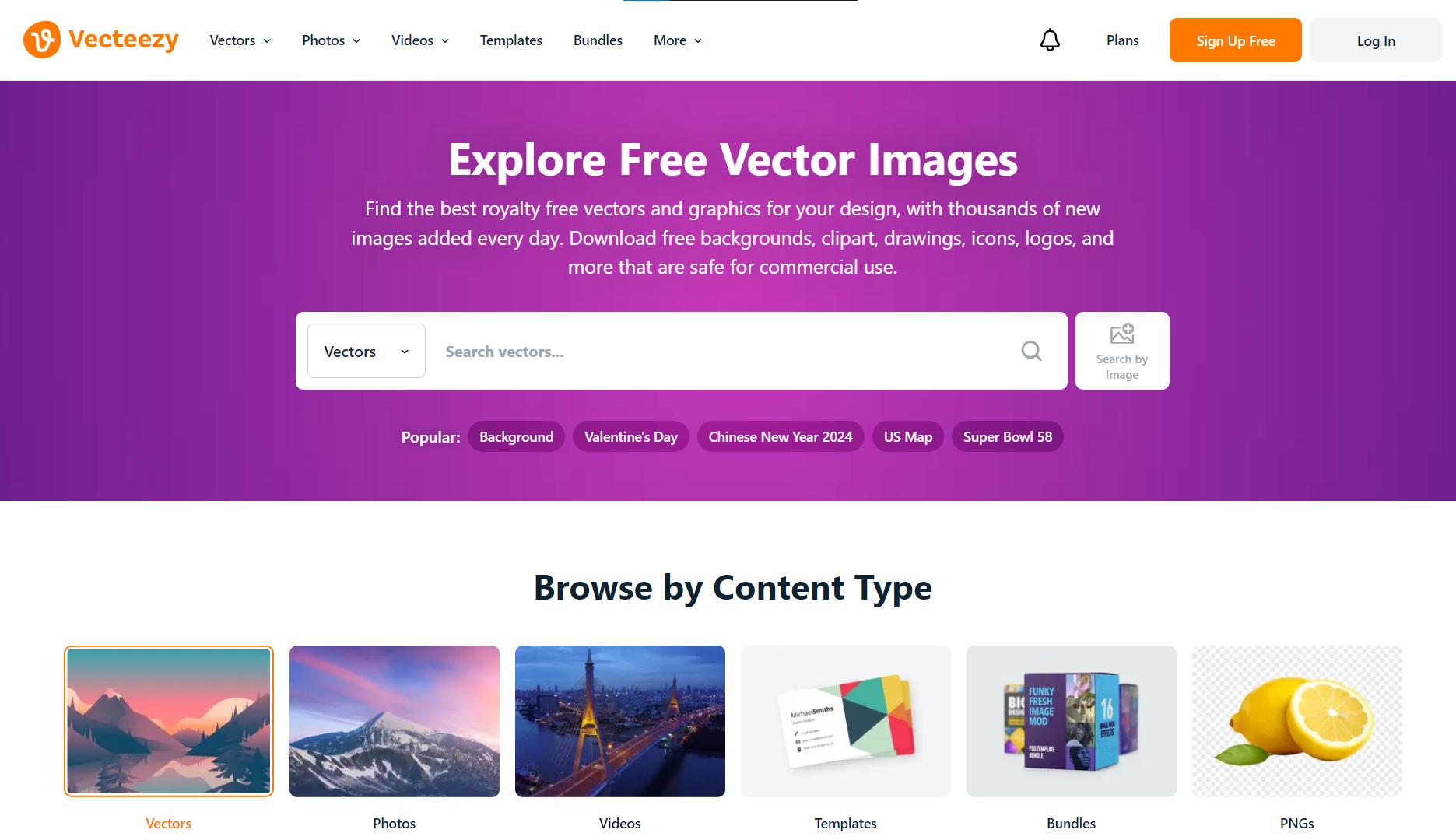The image is a screenshot of the homepage of the Vecteezy website. Positioned at the top left is the website's logo, "Vecteezy." Adjacent to the logo is a navigation bar with various tabs labeled "Vectors," "Photos," "Videos," "Templates," "Bundles," and "More." 

Central to the page is a prominent heading that reads, "Explore Free Vector Images." Below this, a subheading elaborates, inviting users to "Find the best royalty-free vectors and graphics for your design, with thousands of new images added every day." It further encourages users to "Download free backgrounds, clipart, drawings, icons, logos, and more that are safe for commercial use."

Beneath the subheading is a search box with placeholder text indicating "Search vectors." Directly below the search box, the webpage features an option to "Browse by Content Type," guiding users to organize their search more effectively.